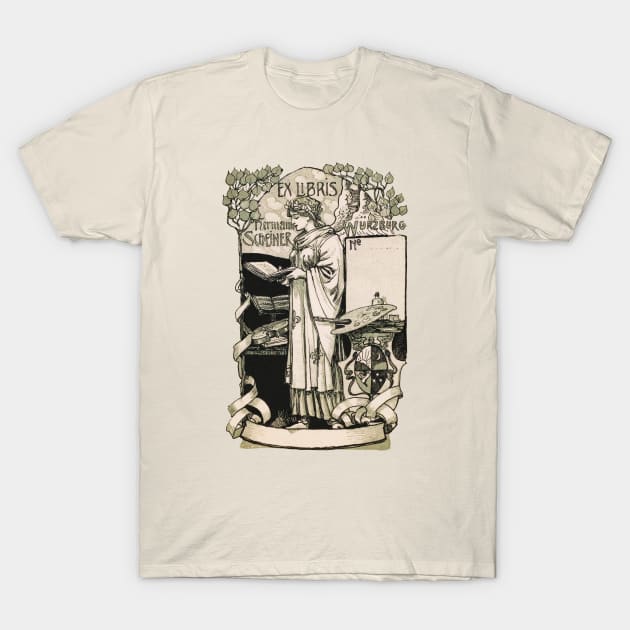This photo showcases a cream-colored, retro-style t-shirt featuring an ornate black print. At the top of the detailed line drawing, the text "Ex Libris" is prominently displayed, reminiscent of old bookplates once common in library books. The central illustration depicts a woman, dressed in a full-length Greek-style gown, intently reading an open book. She stands amidst an intricate setting: a bookshelf to her left, a painter's easel to her right, and decorative ribbons and vines framing the scene. Below her, a blank horizontal banner adds to the vintage aesthetic. Though much of the additional text under "Ex Libris" is blurred and challenging to decipher, "China" and "Wartsburg" can be made out. The photo, taken against a professional white backdrop, highlights the t-shirt's careful detailing, despite its low resolution.